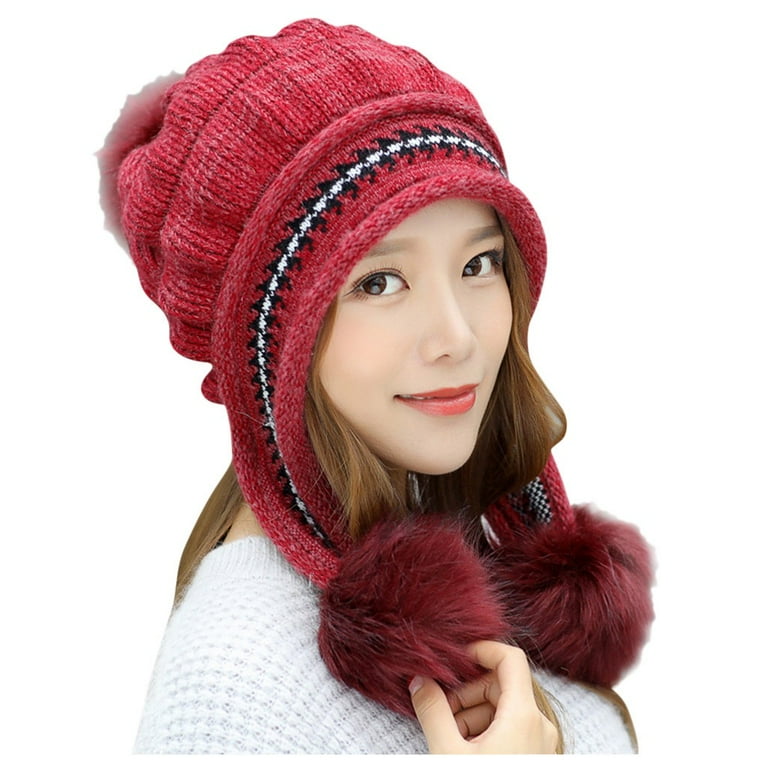The photograph shows a beautiful young Asian woman, likely between the ages of 14 and 20, smiling warmly at the camera. Her lightly tinged red lips hint at subtle lipstick, complementing her pale, nearly translucent white skin. Her large brown eyes gaze directly at the camera, despite her face being slightly turned, giving a three-quarters view. Her light brown, almost blonde hair is framed by a large, red, knitted winter hat adorned with fluffy pom-poms and intricate black and white stitching along the brim and tassels. The hat's furry extensions cascade down the sides of her face, accentuating its cozy, bulky design. She wears a white knitted sweater, with one hand gently caressing a pom-pom, adding to the serene and inviting atmosphere of the image.